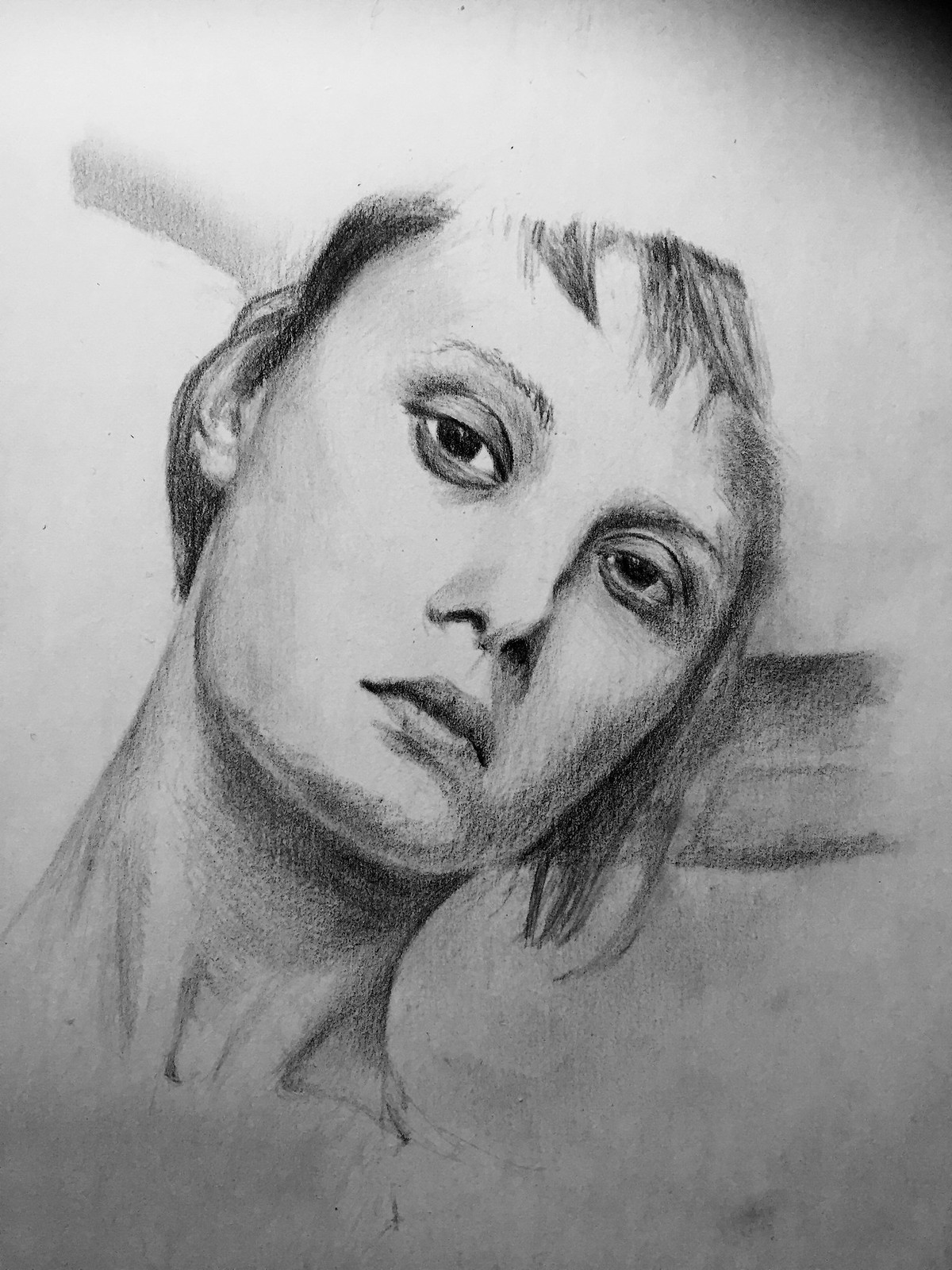The image is a meticulously detailed pencil sketch of a woman, drawn on a pristine white sheet of paper. In the upper right-hand corner, the shading intensifies almost to a deep black, creating a compelling contrast. The woman's face, positioned centrally, exhibits a slight tilt of the head, adding a hint of dynamic motion to the composition. She has short, straight hair rendered in a darker shade, framing her features. Her dark, heavy-lidded eyes convey depth and intensity. Her arms are positioned behind her head, offering an open view of her face and emphasizing her long, well-defined neck where the muscles are distinctly accentuated. The right side of her face is more heavily shaded, enhancing the three-dimensional effect. The woman’s closed lips and serious expression add a contemplative or solemn mood to the portrait.